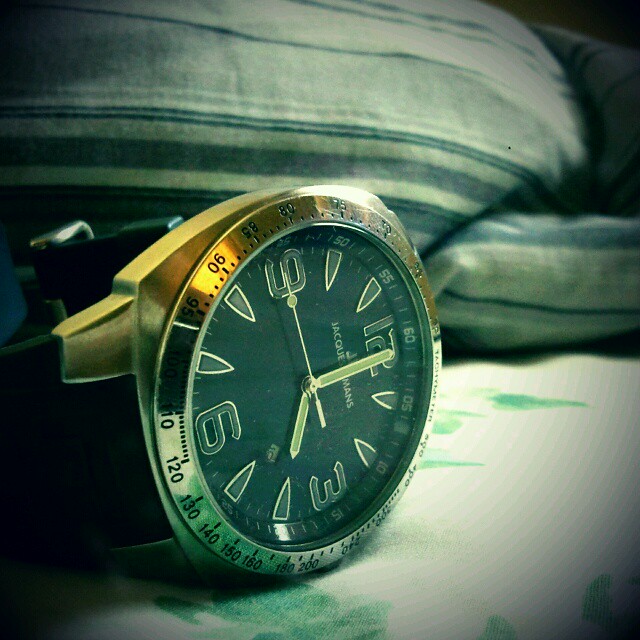The image depicts a large-faced wristwatch placed on a white sheet adorned with green leaves, possibly on a bed. The watch features a prominently large black face with gold-outlined hands and numerals, giving off an elegant, refined look. The main numbers on the watch - 12, 3, 6, and 9 - are clearly visible in gold, along with additional smaller markers. Around the edge of the watch face, a circular gold rim displays numbers like 90, 120, 130, and 140, possibly indicating compass or additional measurement features.

The brand on the watch appears to be "Jackie Mann's" or a similar-sounding name, as partially visible letters "J-A-C-Q-U-E... M-A-N-S" suggest. The hour hand is positioned around the 4 while the second hand rests on the 9. The watch is complemented by a black wristband and an overall sophisticated gold base. Adjacent to the watch, there's a green and cream-colored striped pillow, adding a cozy, intimate ambiance to the setting.